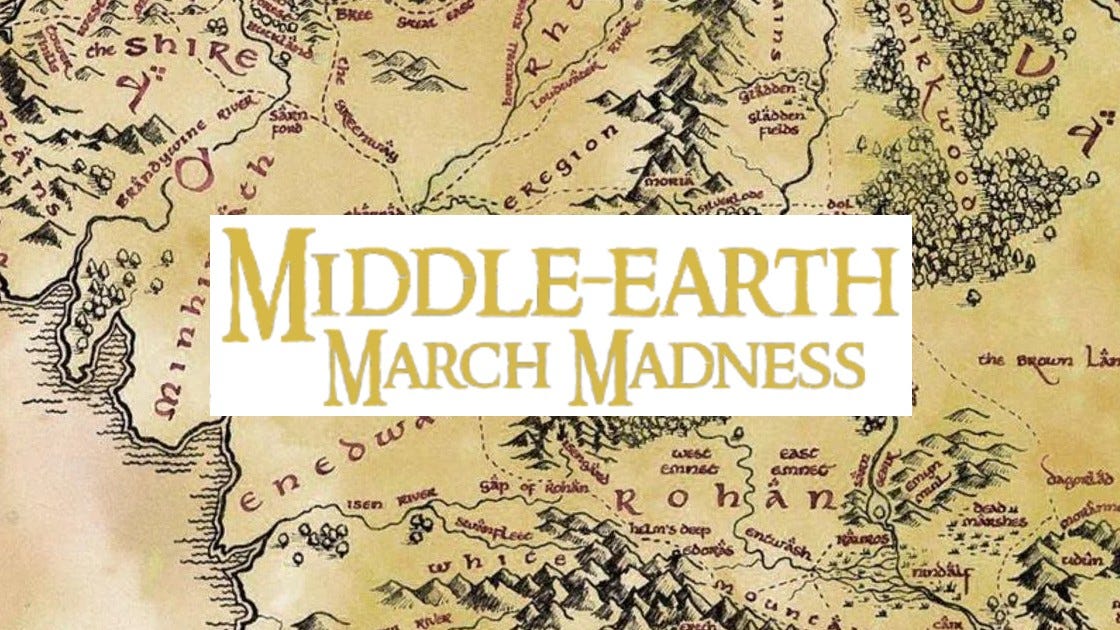The image depicts a detailed, hand-drawn map of Middle-Earth, featuring an old-fashioned style reminiscent of Tolkien's The Lord of the Rings and The Hobbit. The map has intricate features such as mountains, hills, and rivers, all delineated in black ink, with certain areas highlighted in red. A prominent white banner with gold lettering spans the center, bearing the text "MIDDLE EARTH MARCH MADNESS." The background of the map is a dark yellow mustard color which gives it an antique appearance.

Key locations such as the Shire and Mirkwood are labeled, with the Shire positioned at the top left and Mirkwood extending vertically across the top right. Despite some of the labels being blurry, other identifiable names include Rohan, located near the bottom of the map, Kirkwood, and Weiss. The banner obscures part of the map, but visible elements include dotted lines indicating roads and solid lines signaling rivers, like the Brandywine River. The overall scene blends a sense of fantasy cartography with an element of modern, playful adaptation through the "March Madness" announcement.